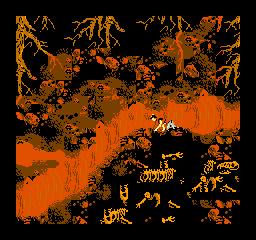This image appears to be a digital illustration, potentially an NFT or a game screenshot, depicting a grim underground scene. The background is entirely black, accentuating the eerie atmosphere. Dominating the scene is a long, red road, textured with maroon lines that slithers off to the left. To the left and right of this road, chocolate brown and red foliage emerges, contributing to the haunting environment.

On the lower right side, skeletal remains, including torsos, spines, and ribcages, stand out in an orangey-white hue against the dark backdrop, indicative of death and decay. Meanwhile, golden foliage and tree-like roots or branches emerge from the top of the image, blending into the darkness.

In the center, three indistinct human-like characters appear to be precariously perched on the road, seemingly on the verge of falling into an ominous red sea, emphasizing the perilous nature of their situation. The low resolution adds to the mysterious and hellish tone of the scene.